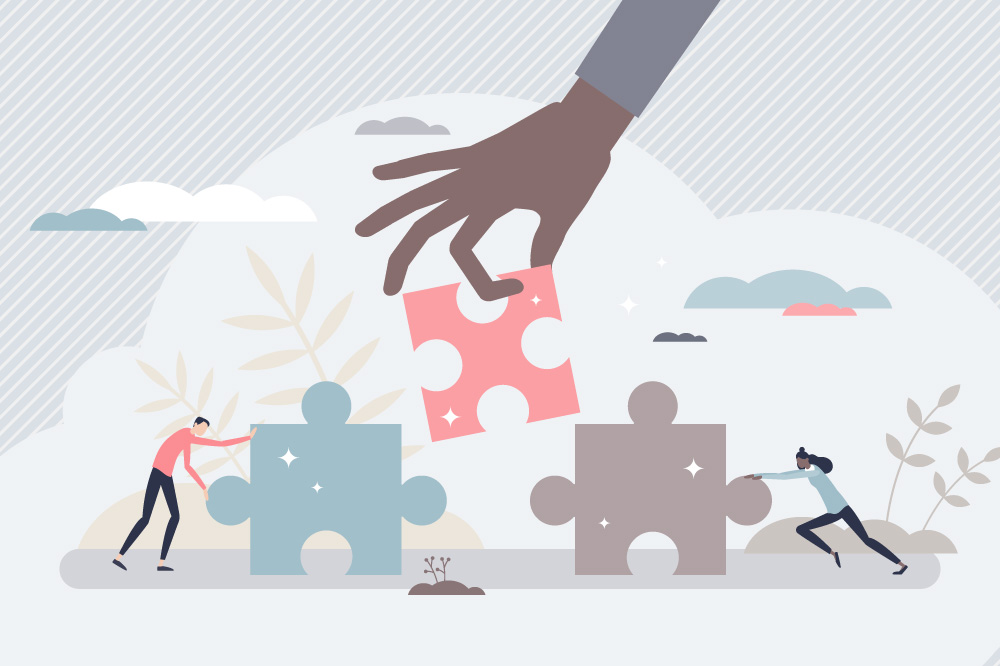The illustrated image shows three puzzle pieces near each other, each adorned with two white stars. On the left, a man with short black hair, wearing a pink shirt and black pants, pushes a teal puzzle piece to the right. On the right, a woman with long black hair, dressed in a blue top and black pants, pushes a grayish-brown puzzle piece to the left. Above and between these pieces, a large dark-skinned hand, emerging from the top of the image and wearing a long sleeve shirt down to the wrist, holds a pink puzzle piece that looks like it would fit snugly between the other two. The overall drawing style is simple and cartoonish, with basic shapes and minimal shading. The background features clouds and various plant silhouettes, adding a serene atmosphere to the scene.